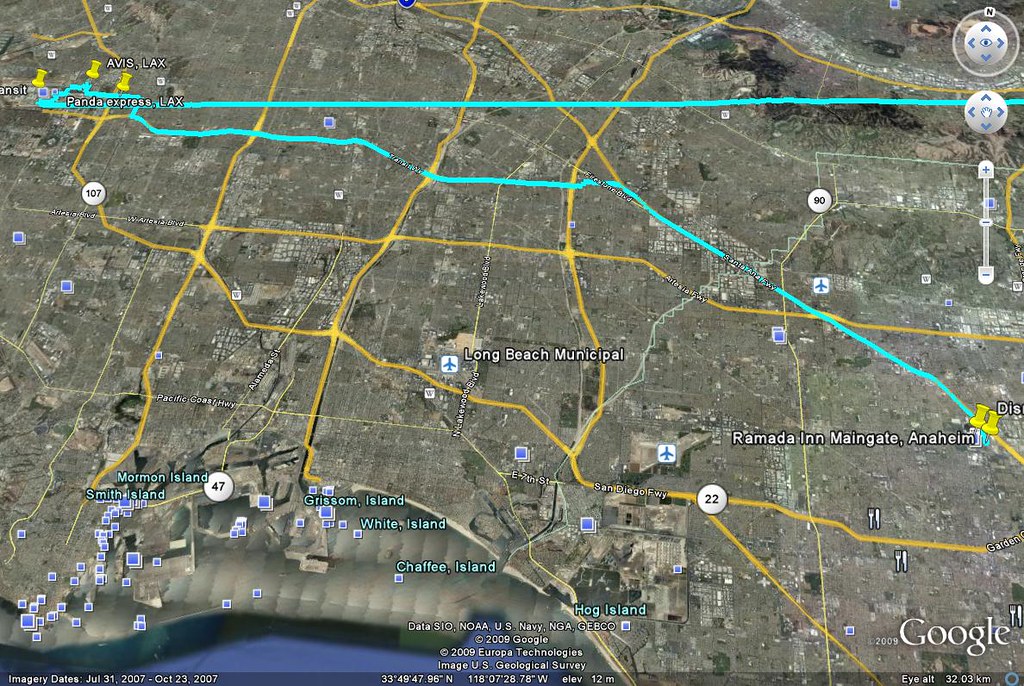The image captures a computer screen displaying an early version of what appears to be Google Maps, with a "Google" watermark located in the bottom right corner. The map features a satellite view with highlighted roads in yellow. Notable landmarks and labels include "Long Beach Municipal Airport," "Ramada Inn," and "Main Gate, Anaheim," while a mention of “Avis Car Rental LAX” indicates the Los Angeles International Airport. Various streets are marked, some with road numbers listed. The map bears a copyright date of 2000, suggesting that it is an older iteration of the mapping service we recognize today. The display overall indicates a simpler and less detailed version of modern digital maps.